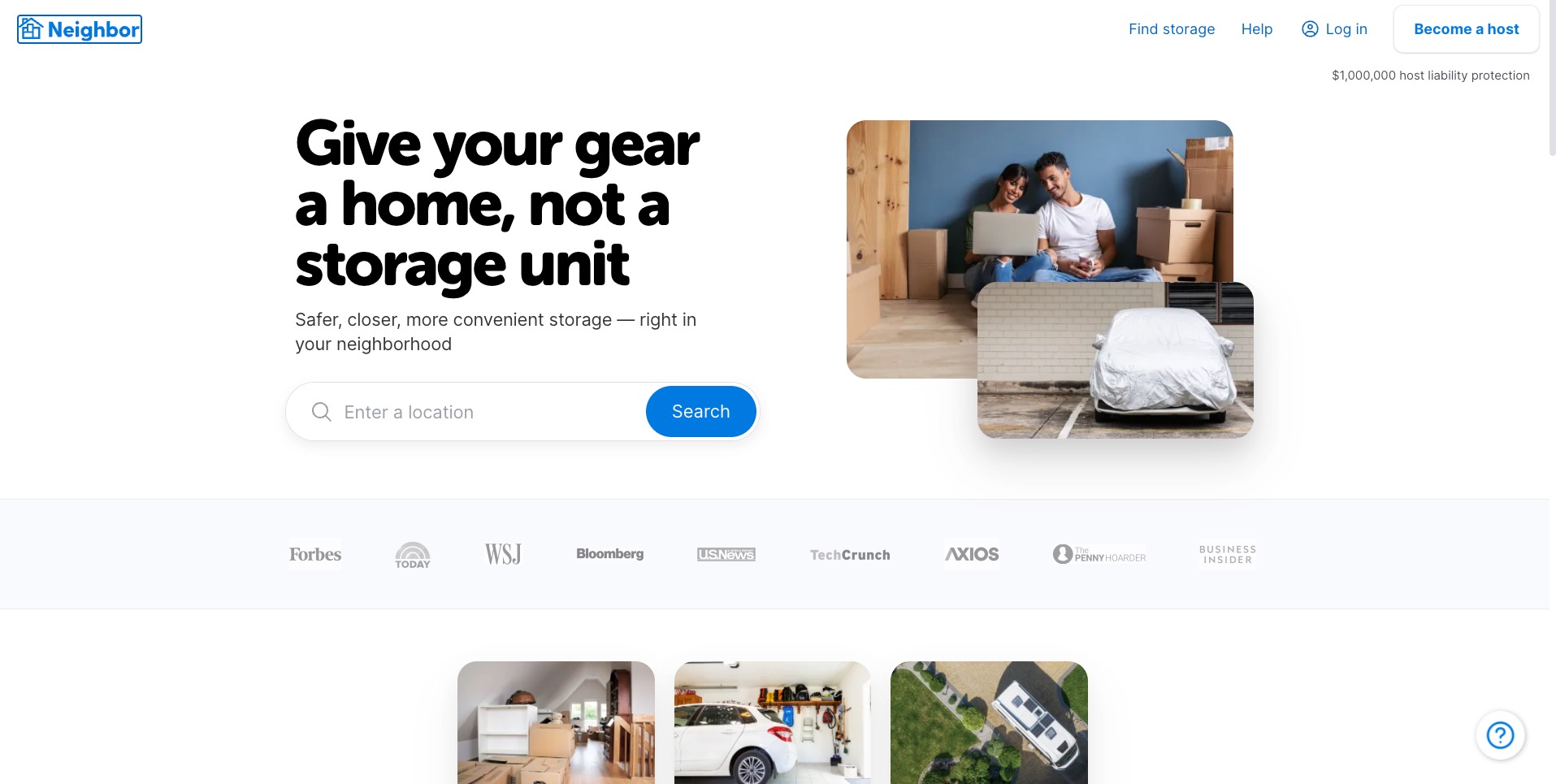The image captures a webpage from a storage-sharing website. In the upper left corner, there is a house icon next to the word "Neighbor," all designed in a blueprint style. At the top right, the navigation menu includes options for "Find Storage," "Help," "Log In," and a prominent "Become a Host" button in a white rectangle.

Below the header, the main tagline reads, "Give your gear a home, not a storage unit," emphasizing the benefits of using neighborhood storage with the phrases "safer, closer, more convenient storage right in your neighborhood." Beneath this, a photograph shows a couple sitting on the floor of a house, surrounded by moving boxes, suggesting they are either moving in or packing up. Adjacent to this image is a picture of a car parked in a spot with a white cover over it.

There is a search area where users can enter a location, accompanied by a blue "Search" button. Dividers showcase endorsements from well-known publications like Forbes, Today, WSJ, Bloomberg, US News, and TechCrunch. At the bottom, additional images depict various home storage solutions around the neighborhood.